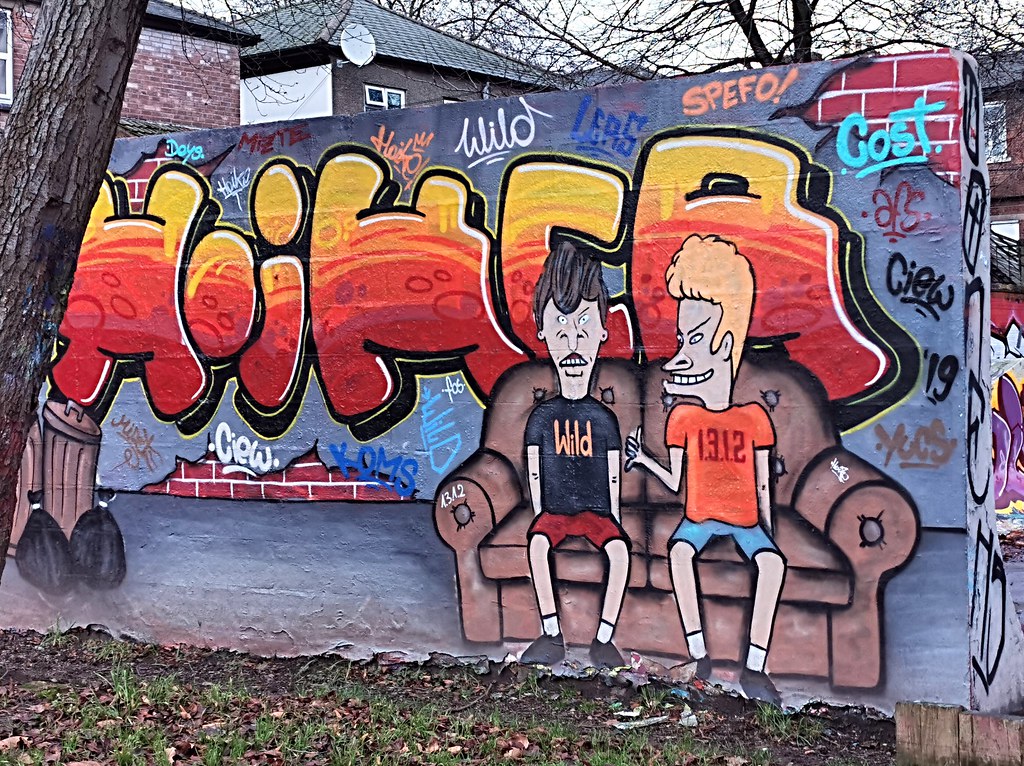In this vibrant piece of graffiti-style artwork, a large wall, possibly adjacent to a housing complex or within a backyard, features a colorful and detailed cartoon image of Beavis and Butthead. The wall's primary hue is blue, adorned with various tags and writings in black, blue, white, orange, and yellow. Prominent graffiti elements include the words 'Wild', 'speco', 'cost', 'crew', and more, with large, somewhat unintelligible orange and yellow letters towering over the rest.

At the center of the scene, the iconic duo sits on their familiar brown loveseat. Beavis, identifiable by his black t-shirt emblazoned with 'Wild', and Butthead, sporting an orange t-shirt that reads '1312', are depicted mid-conversation. Their detailed expressions capture the essence of their animated personas.

To the left of the image stands a grand oak tree, adding a touch of nature to the urban canvas, while a couple of trash cans are visible to their right, blending seamlessly with the backdrop. The mural backdrop comprises older brick houses, indicating a subdivision, enhancing the artwork's realism. The level of detail and artistic talent behind this graffitied wall makes it a standout piece within its environment.